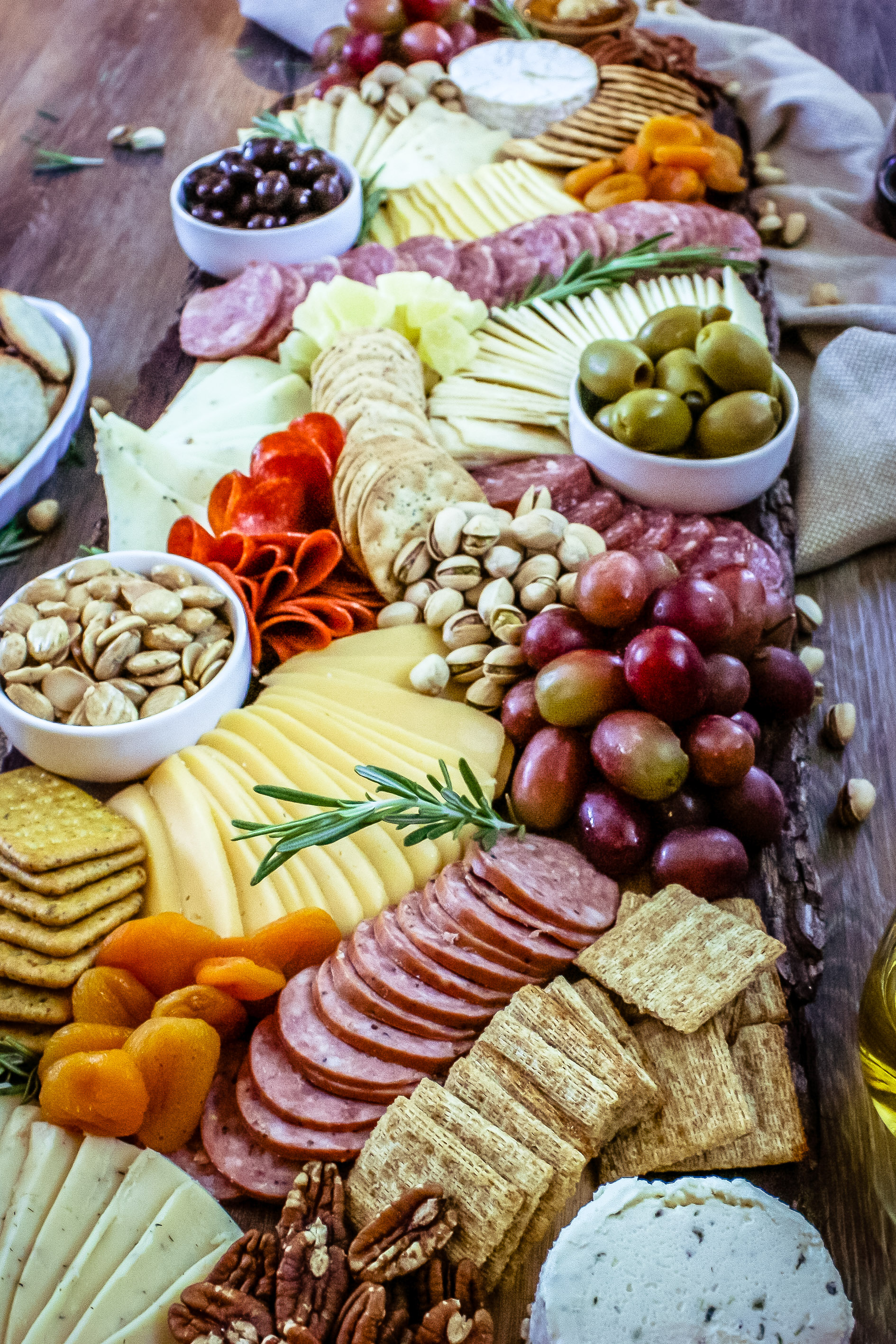The image depicts a zoomed-in view of an elaborate charcuterie board placed on a rustic wooden table. The board is densely packed with an assortment of foods, artfully arranged for easy grazing. Starting from the bottom left, there are slices of various cheeses, including white cheese, Swiss, and provolone. Adjacent to the cheese are pecans and a soft cheese or pate. Moving upwards, a selection of crackers, such as wheat thins and triscuits, can be seen next to neatly stacked slices of salami and pepperoni, the latter often curled for a decorative touch. Above the crackers, a variety of fruits like grapes and possibly dried apricots and dried pineapple add a sweet element to the spread. 

In the center, small white bowls contain green and black olives, surrounded by clusters of nuts including pistachios and walnuts. The upper portion of the board features more cheeses, likely including blue cheese, and additional types of sliced meats, such as ham. A round serving of brie is also noticeable. The diverse assortment of crackers, cheeses, meats, fruits, and nuts creates a visually appealing and tempting charcuterie board. Flanking the board, there is a woven tablecloth or sackcloth and a bowl of bread, adding to the rustic aesthetic. Overall, the image highlights a sumptuous spread, ideal for indulgent snacking and sharing.